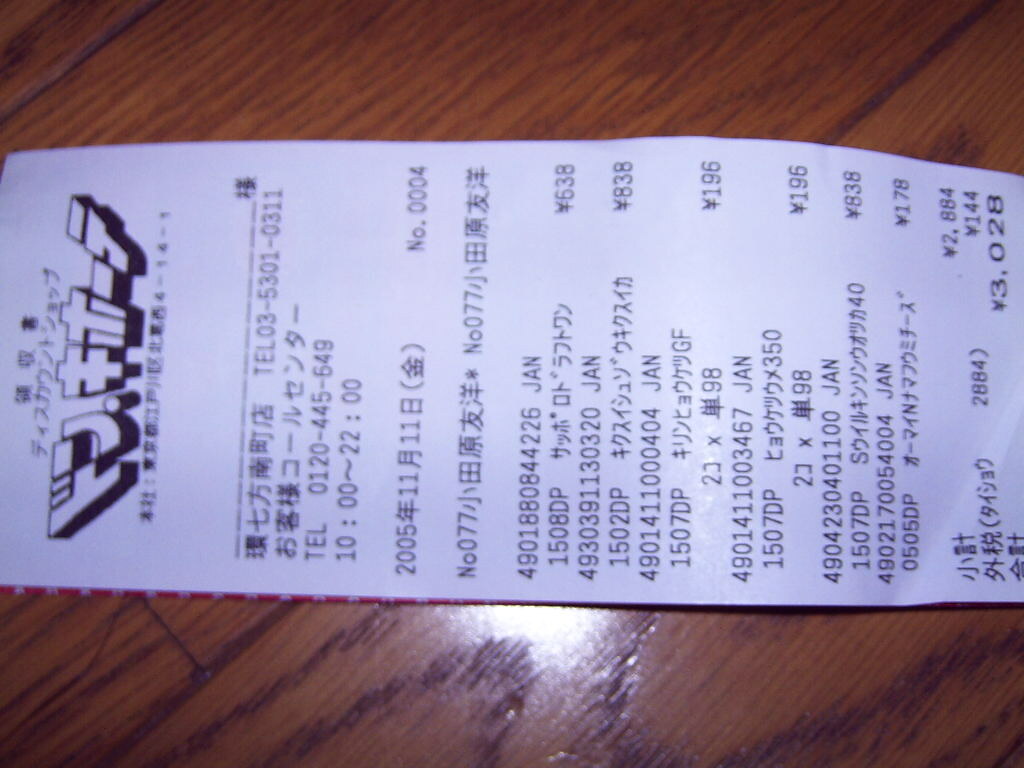This image captures a paper receipt, likely of Japanese origin, laid sideways across the center of a reddish-brown wooden table with a visible plank pattern. The table features subtle, darker stripes running through its lighter wood. The receipt, made of white paper, is a long, rectangular shape and oriented on its side, making it challenging to read. The upper portion of the receipt displays bold Japanese characters with flared edges, while the rest is filled with detailed black text and numbers. Among the readable information is a telephone number, TEL 0120-445-649, and potentially a total amount of 3.028, though it's unclear if this is in Japanese currency. Despite the language barrier, the receipt’s intricate, foreign-style characters and numerals offer a glimpse into its origin.